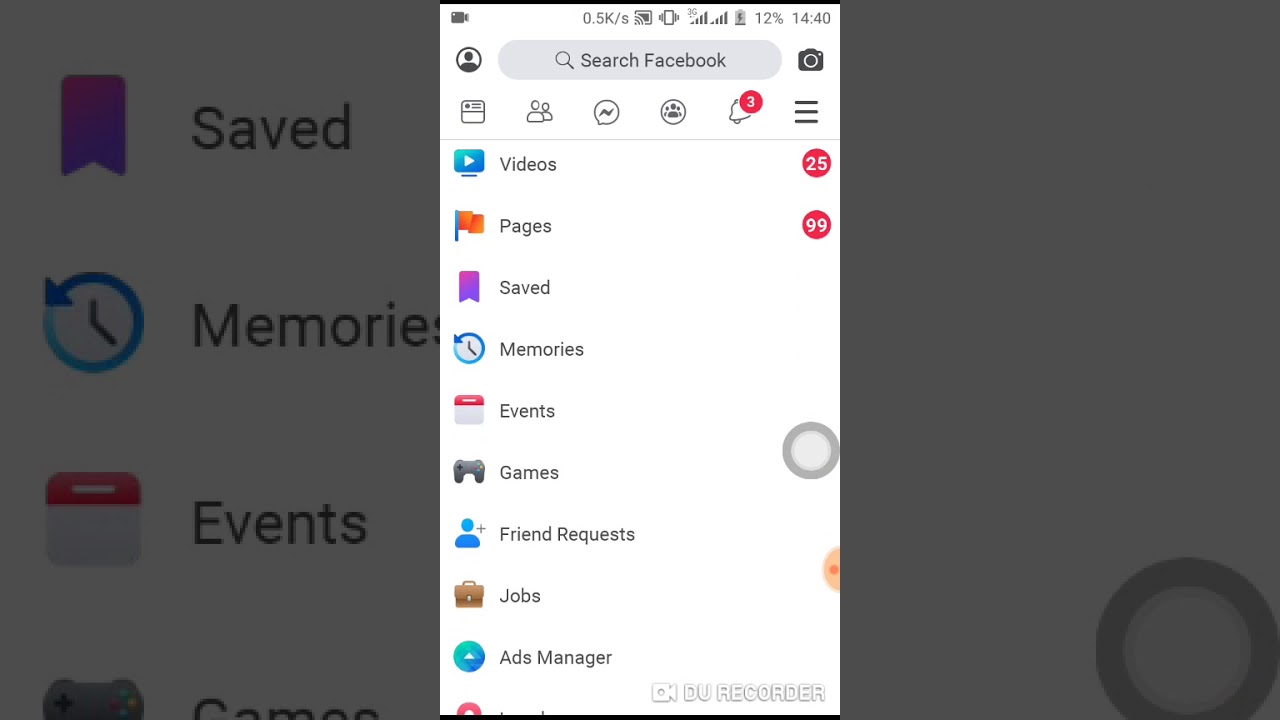The screenshot features the interface of a mobile application, predominantly showcasing Facebook's navigation menu. The background is subdued with a grayish tint, making the large icons in the foreground particularly prominent. At the top center of the image, there is a search bar labeled "Search Facebook," which suggests the user can enter queries directly.

Below the search bar, there are several sizable icons accompanied by text to their right, organized in a vertical layout:
1. A monitor icon with the text "Videos," marked with a play button.
2. A flag icon labeled "Pages."
3. A purple bookmark symbol, accompanied by the text "Saved."
4. A clock icon indicating "Memories."
5. A calendar icon labeled "Events."
6. A PlayStation controller icon titled "Games."
7. A simple round circle emblem representing a person's head and shoulders, associated with "Friend Requests."
8. A briefcase icon indicating "Jobs."
9. A triangle symbol labeled "Ads Manager."

Above this section, beneath the search field, there is a row of basic black and white icons denoting different functionalities:
- A calendar.
- Two people standing next to each other.
- A speech bubble with a lightning bolt.
- A trio of people in a circular arrangement.
- A bell icon with a notification bubble showing the number three.

Further down, within the "Videos" icon, there is a red notification circle displaying the number 25, and adjacent to the "Pages" icon, there's another notification bubble showing the number 99.

This meticulous arrangement of icons and notifications provides quick access to various Facebook features, ensuring users can easily navigate through different sections within the app.